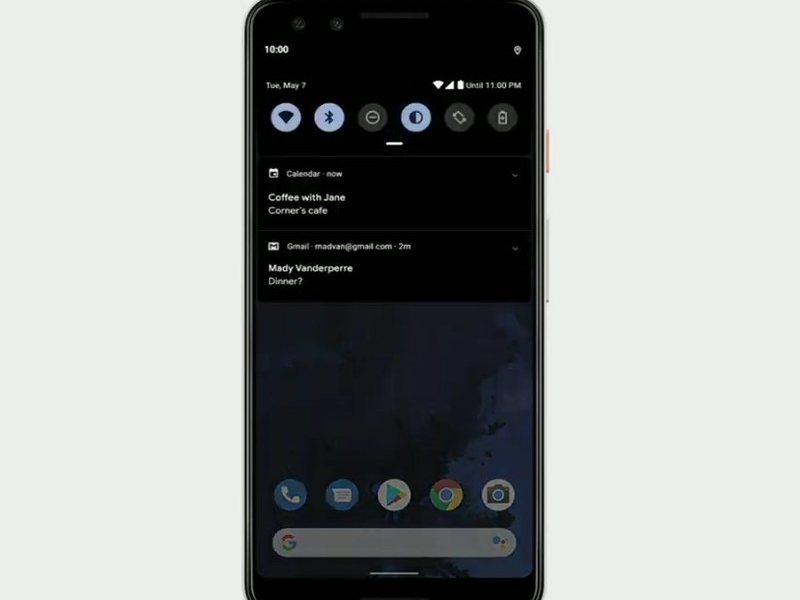A sleek black cell phone is centered against a light gray background. The device displays a detailed interface:

- **Top of the Screen:**
  - The time reads **10:00**.
  - Below the time, it shows **Tuesday, May 7th**.
  - On the right-hand side is a vertical, fully-charged battery icon in white.

- **Middle Section:**
  - Features a horizontal row of status icons: 
    - A **blue circle**.
    - Another **blue circle** next to it.
    - A **black circle**.
    - A blue circle with a black half overlapping a light blue background.
    - **Two black circles** following it.

- **Main Content:**
  - **"Calendar Now"** is written prominently.
  - Below, in white text: **"Coffee with Jane"**.
  - Followed by the location: **"Corners Cafe"**.
  - An alert from **Gmail**, stating:
    - **"Two minutes ago"** from the user **Mady Vanderpere**.
    - The message preview reads **"Dinner?"**.

- **Bottom Section:**
  - Mostly black with a hint of dark blue on the right side, resembling the beginning of a map.
  - The bottom edge showcases prominent cell phone widgets:
    - A **phone icon** within a blue circle.
    - A **Google arrow** in a white circle.
    - The **Google Chrome** icon depicting its iconic red, yellow, green outer colors, and a blue inner circle.
    - Lastly, the ever-present **Google search bar** spans across the bottom.